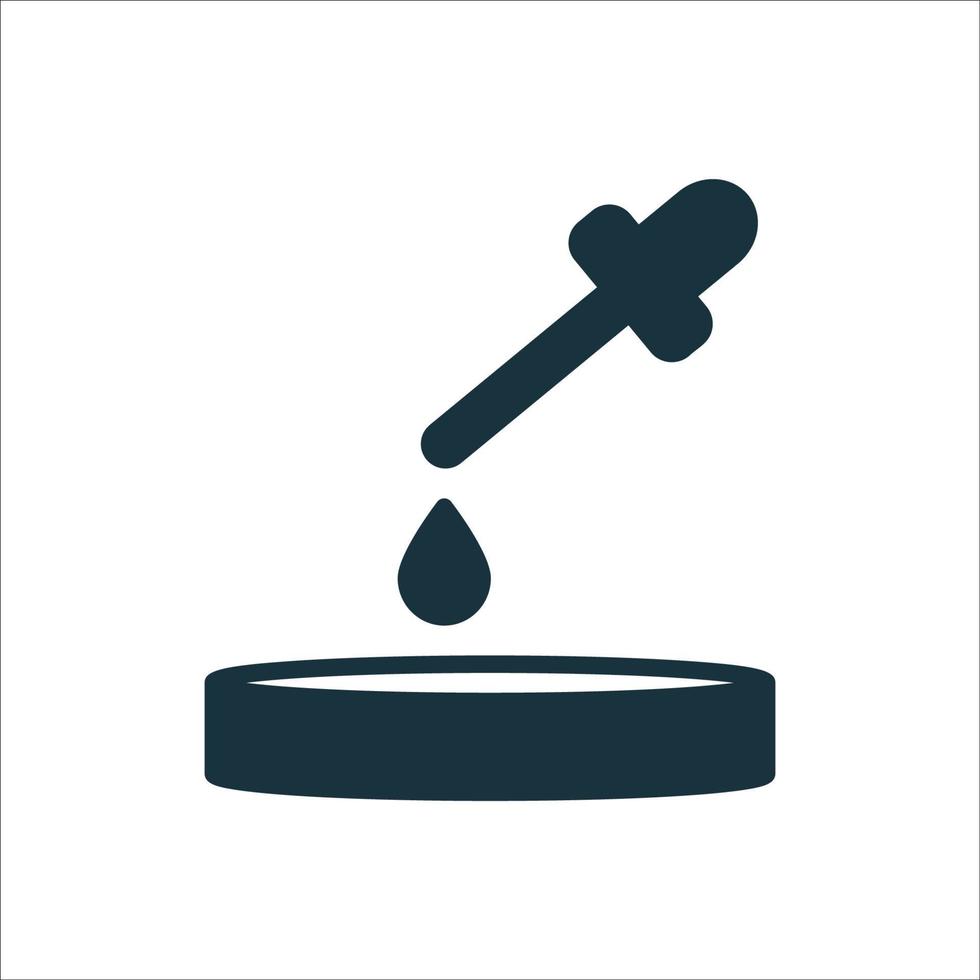The image is a simple, minimalist design featuring a navy blue dropper with a droplet falling into a shallow dish below it. The three objects—the dropper, the droplet, and the dish—share the same deep dark blue color, contrasting sharply against a pure white background. The dimensions of the image are square. The dropper, resembling a miniature turkey baster with a tube on the left and a rubberized handle on the right, dispenses a sizeable droplet of liquid, which is captured in mid-air, just about to land in the dish. There is no hand present, making the dropper appear as if it operates autonomously. The overall aesthetic is simple and could be likened to an emoji or a computer graphic.